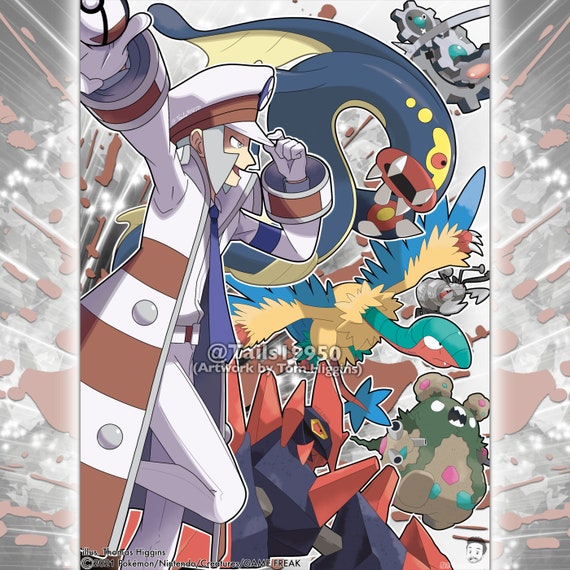This captivating anime-style poster appears to be an advertisement or artwork related to Pokemon. Dominating the left side, a central figure dressed in an elaborate and stylish outfit draws attention. This character is attired in a completely white ensemble accented with brown stripes, including a long trench coat, a captain’s hat with a brown stripe, white top and pants, and a purple tie. Striking a dynamic pose, the figure adjusts the tip of their hat with their left hand while extending their right hand, which seems to cradle a ball-like object.

To the right of this character, a vivid array of fantastical creatures fills the background, reminiscent of Pokemon. Among them is a large, blue-and-yellow creature that resembles a bird with a turtle-like head and animatronic features. Beneath it, a vibrant bird adorned with green, red, yellow, and blue colors spreads its wings majestically. In the lower right corner, a small, menacing green and light beige monster with sharp teeth and white eyes stands with its mouth agape. 

An additional character, resembling a green mouse with large ears, adds to the whimsical scene. The composition's color palette consists of subdued yet diverse hues, contributing to the overall artistic charm. A copyright note in the center reads "ATTAILSL9950, artwork by Tora Higgins," highlighting the creative genius behind this detailed and imaginative piece.